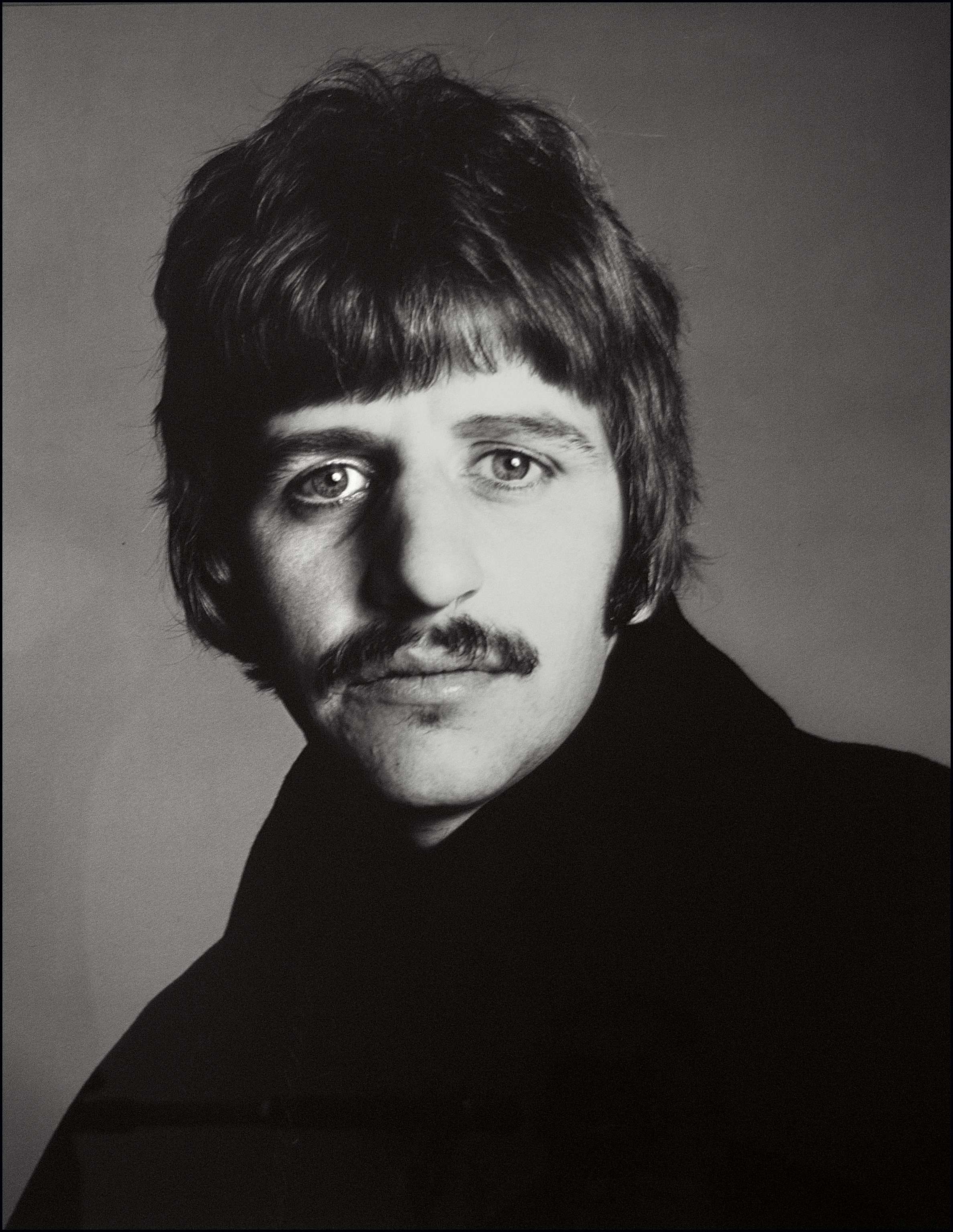This black and white photograph captures a young white male, possibly from the 50s or 60s, looking directly at the camera. The man stands centered against a plain gray background, giving the image a professional studio feel. He has dark, relatively short hair styled into a voluminous top with blunt bangs and long sides, resembling sideburns, and likely brown in color. His bushy mustache and a small patch of hair under his bottom lip add to his distinctive appearance. His eyes, which appear droopy, would probably be blue if the photo were in color. He is dressed in a large black coat with a thick, high collar, which could be a turtleneck or an overcoat. The overall composition is simple yet evocative, highlighting the detailed textures of his features and attire.